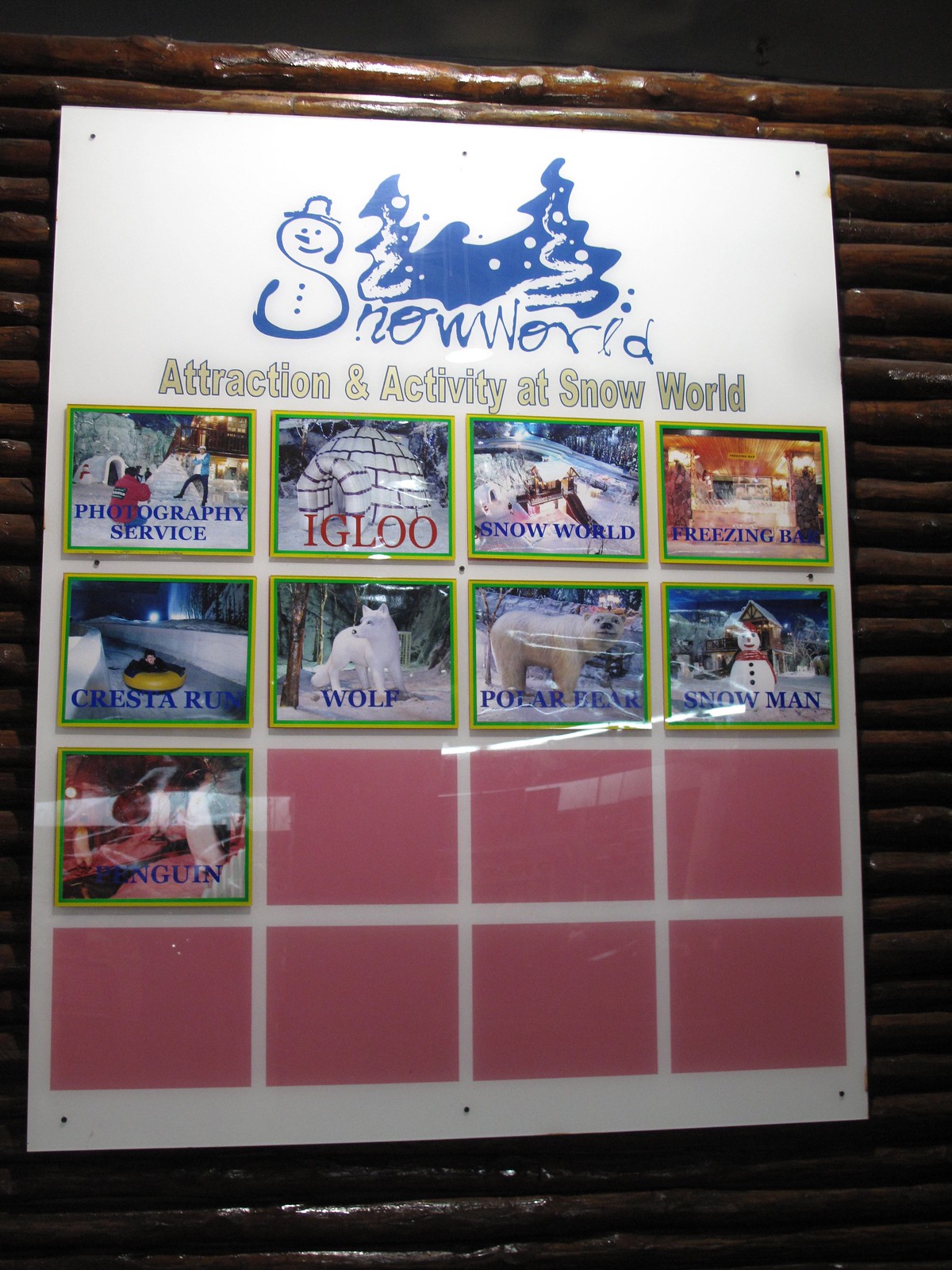In this dimly lit image, we see a central information board, prominently displaying the text "Snow World" in blue letters against a light background. The "S" in "Snow World" cleverly incorporates an illustration of a snowman. Positioned on a background made of horizontally stacked dark brown, shiny sticks, the board appears to be hanging against a bamboo-like wall. 

The top portion of the sign lists various attractions and activities at Snow World, organized into 16 squares. Seven of these squares, adorned with photos or icons, represent: Photography Service, Igloo, Snow World, Freezing Bar, Crest Run, Wolf, Polar Bear, Snowman, and Penguin. The remaining nine squares at the bottom are distinctly red but remain blank, neither containing images nor text. A visible reflection hints at a protective glass cover over the board. 

The colors present in the scene include black, brown, white, blue, gray, green, red, and pink, which enhance the overall visual appeal of this indoor setting, presumably within an amusement park.